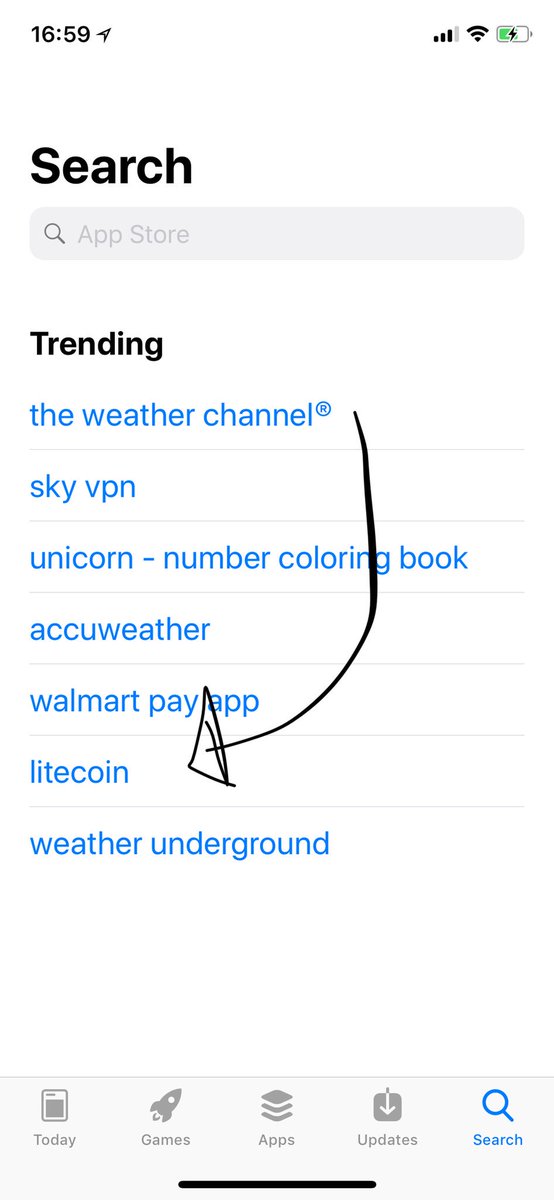Here is a cleaned up and detailed caption for the image:

---

This vertical portrait screenshot captures a phone screen displaying the App Store's search page. The status bar at the top shows it is 16:59, with 3 out of 4 service bars, a full Wi-Fi signal, and a battery about half full and charging. Just below the status bar, a white background features black text that reads "Search" alongside the App Store search box. Underneath, a 'Trending' section lists popular apps in blue text: The Weather Channel, Skype VPN, Unicorn, Number Coloring Book, AccuWeather, Walmart Pay App, Litecoin, and Weather Underground.

Notably, an arrow is hand-drawn in black, pointing towards "Litecoin" in the list, hinting at the primary focus of the screenshot. At the bottom of the screen, navigation buttons for Today, Games, Apps, Updates, and Search are visible. Given the emphasis on Litecoin, it appears the screenshot is intended to guide someone on how to find and download the Litecoin app from the trending section of the App Store. Without additional context, the exact purpose remains speculative, but the focus is evidently on highlighting the Litecoin app.

---

Hope this meets your needs!